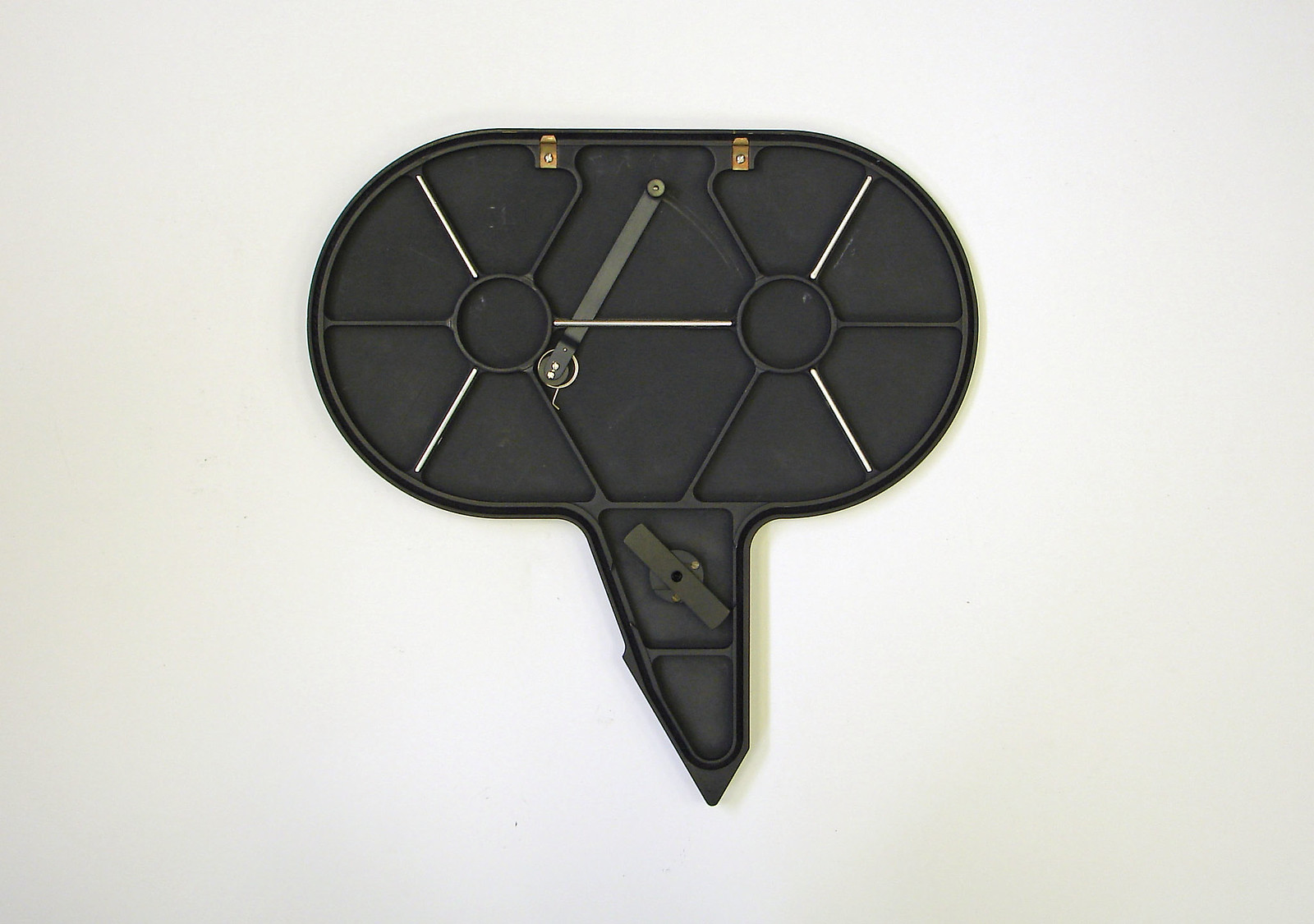The object depicted in the image resembles the shape of a speech bubble typically seen in comics or cartoons, with a rounded main section and a tapered "tail" extending from it. It is not a speech bubble, however. The primary structure consists of a large, oval-shaped base featuring two prominent circular components—one positioned on the right and the other on the left. At the center, a small metal tool appears to be secured under a slim metal bar, potentially held in place by a pin. This metal tool looks somewhat like a tiny belt with a silver piece hanging from either the top or the bottom. Below the oval, in the "tail" portion of the supposed speech bubble shape, there is another circle intersected by a bar. The entire object is divided into sections, many of which are triangular in shape. The color of the object is gray. Despite the detailed observation, the exact purpose or identity of this object remains unclear.